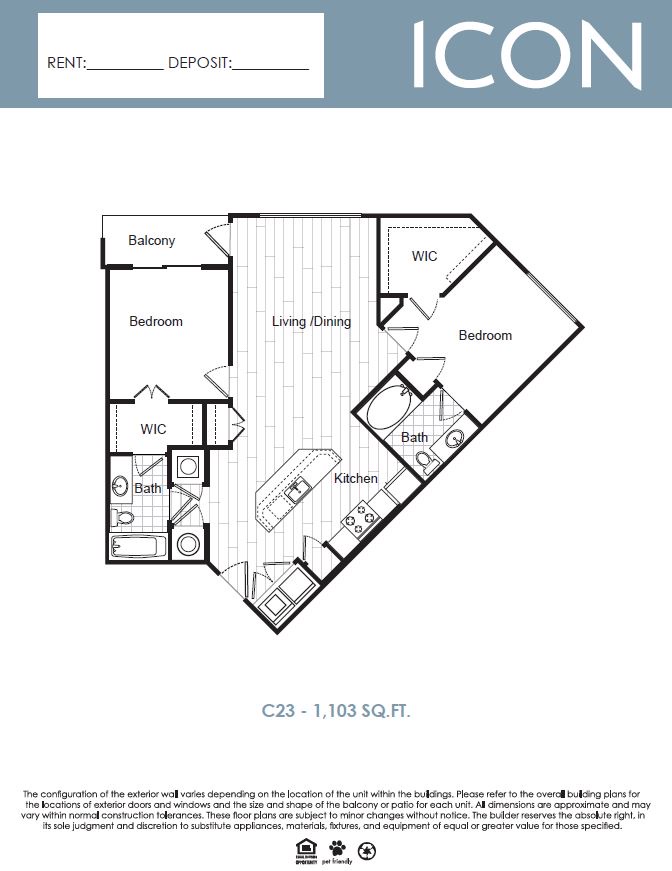This image depicts a detailed blueprint of an apartment complex. The design incorporates a combined living room and dining room area, seamlessly connected to the kitchen. The layout features two spacious bedrooms and a single bathroom. The thoughtfully organized blueprint offers a clear vision of the apartment's functional and communal spaces, delivering a cohesive and practical living environment.